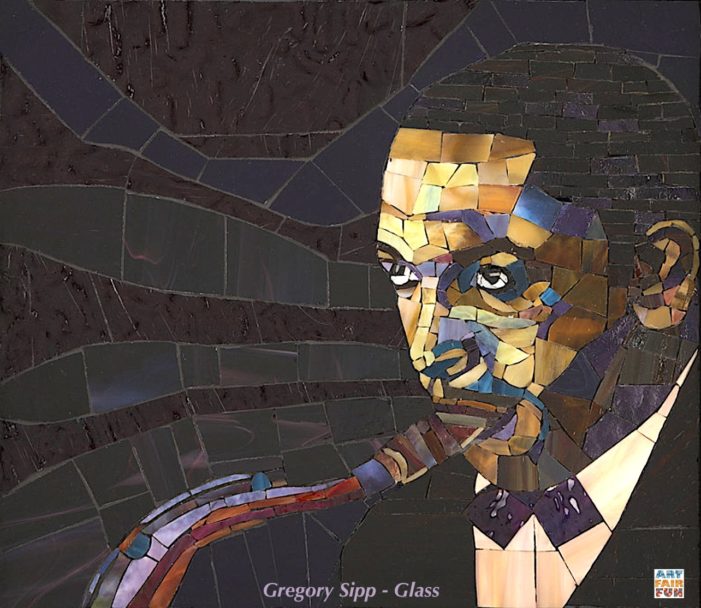This piece of art is a detailed mosaic collage, primarily crafted from various materials such as glass, paper, and possibly metal, with a vivid and textured effect. Dominating the right side of the image is the portrayal of an African man with close-cropped dark black hair and distinct dark skin, accentuated by panes in bright hues like blue, orange, and purple for heightened depth. The man, attired in a black suit jacket, white shirt, and purple bow tie, gazes toward the top left of the image. Emerging from his mouth is a burst of colored glass shards in shades of purple, red, orange, and brown, suggesting a flowing vibrancy, interspersed with small blue button-like elements, hinting at a musical instrument, potentially a saxophone, that lends an auditory illusion to the visual. The intricate background features swirling, dark-toned glass panes in black, navy blue, and dark green, creating a dynamic contrast. Centered at the bottom of the image are the words "Gregory Sip-Glax," accompanied by a small multicolored logo in white, blue, orange, and red positioned in the bottom right corner, which adds a finishing touch to this captivating mosaic artwork.